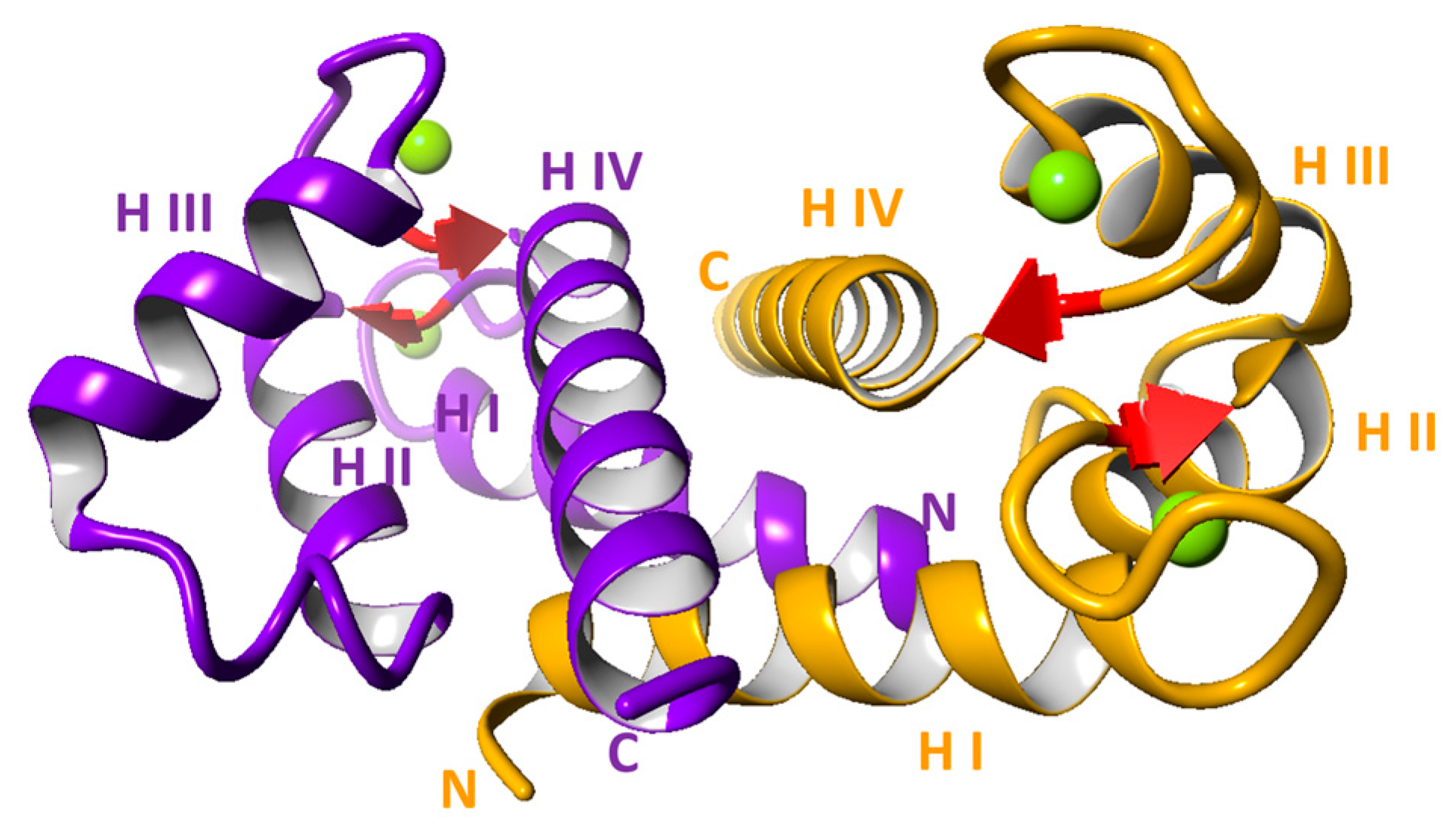The image is a scientific illustration featuring a series of spiral-shaped forms and text against a white background. The spirals, which resemble ribbons, are primarily in shades of purple, yellow, and gold, with some transitions between these colors. There are also red arrows pointing in various directions throughout the diagram. The spirals vary; some have their ends pulled out slightly and some morph into tubes filled with color. Scattered across the image are various pieces of text in both purple and yellow, including "H-I-I-I", "H-I-V", "H-I-I", "H-I", "N", and "C". The layout appears to be complex, resembling a flowchart, with these texts positioned at different points within the illustration.